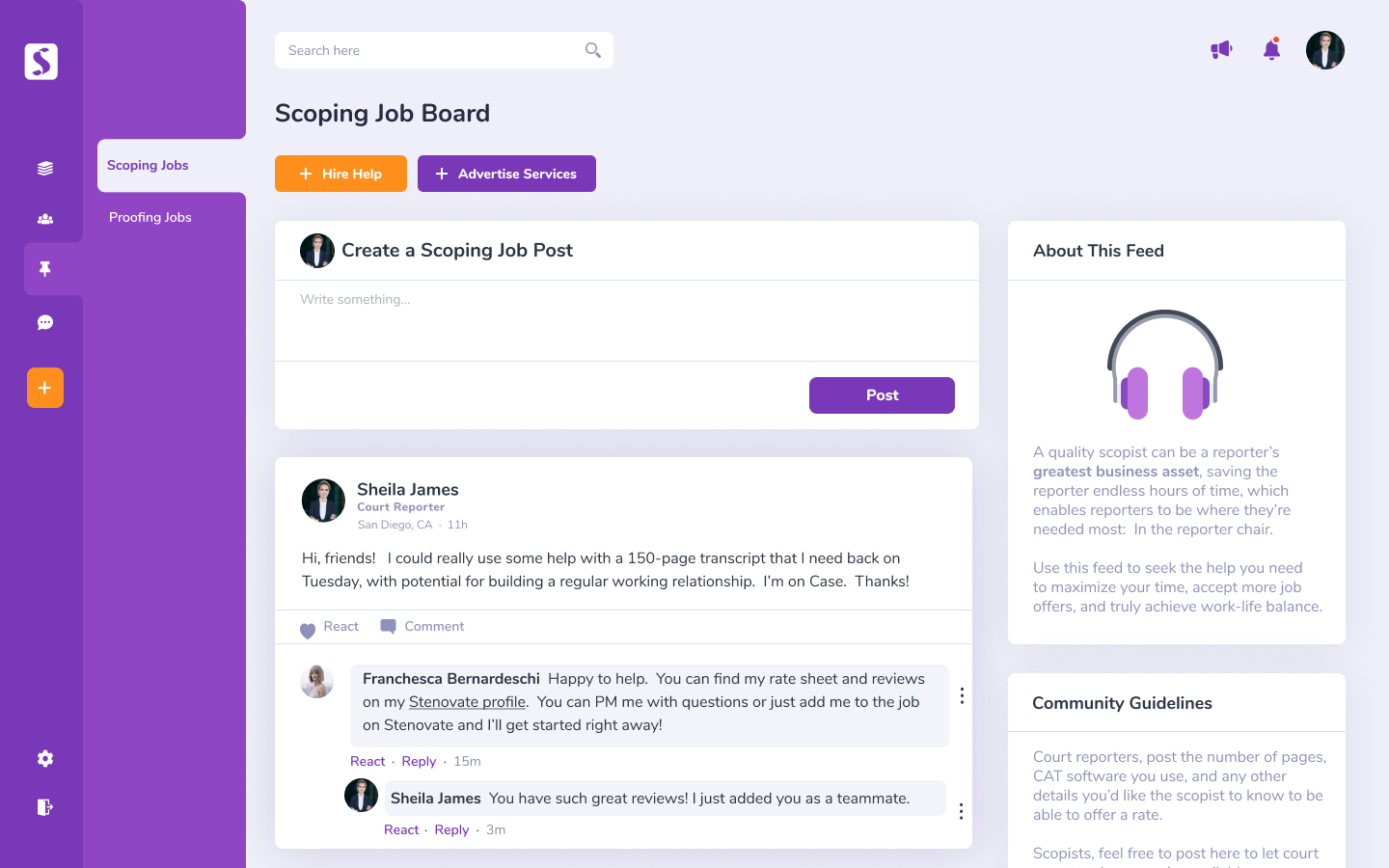In this image of a job board interface, the layout features a left vertical menu encapsulated in a purple box. This box spans from the top to the bottom of the screen, with the left portion of the box shaded a darker purple. At the top of this darker section, there is a white square with a centrally positioned purple 'S'. Beneath this square, four vertically aligned icons are displayed, followed by a yellow box containing a white plus sign. At the bottom of the menu, a gear icon and another white icon are visible. Notably, the pin icon is selected, indicating its active status.

The menu includes two primary options: "Scoping Jobs" and "Proofing Jobs." Moving to the right-hand side, which forms the main window of the interface, the section is headed with the title "Scoping Job Board." Directly below this title are two buttons: one for "Hire Help" and the other for "Advertise Services." Below these buttons lies a prominent white box labeled "Create a Scoping Job Post," accompanied by a text input box for users to enter job details. To the bottom right of this section is a vivid purple button labeled "Post."